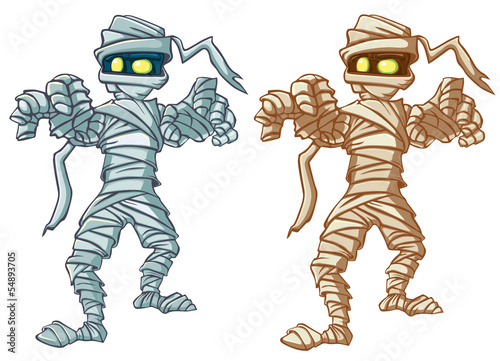The image is a detailed drawing of two cartoonish mummies advancing towards the viewer against a white background. The mummy on the left has a bluish-gray hue, while the one on the right is adorned in tan and light brown tones. Both figures are meticulously wrapped in tattered, jagged bandages from head to toe, with some bandages trailing off their arms and heads, giving a sense of dishevelment. Their large, glowing yellow eyes dominate their faces, contrasting vividly against dark backgrounds—teal for the bluish-gray mummy and brown for the tan mummy. The eyes are peculiarly shaped, with one eye being round and the other egg-shaped and slanted. With arms extended forward and their right legs stepping out, they emanate an eerie sense of motion as if coming towards the viewer, reminiscent of a scene from a horror movie or animated thriller. Their posture, resembling a martial arts stance, adds an element of dynamic tension to the composition. A text reference on the side of the image reads "Adobe stock" followed by a number, marking the image's source.